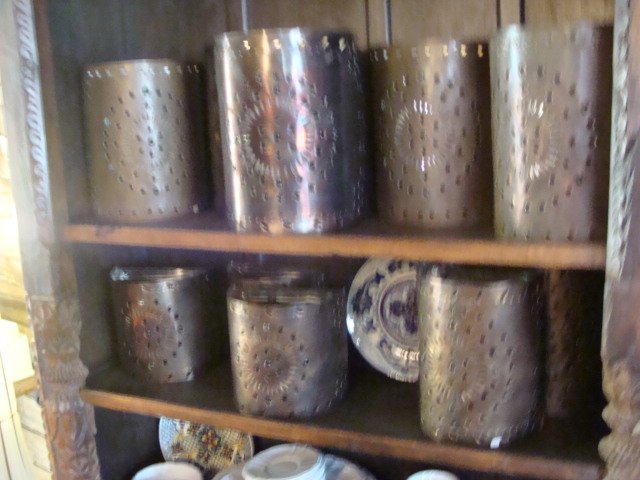This out-of-focus photograph depicts a carved wooden bookcase with paneling in the background, featuring two shelves lined with cylindrical metal candle holders. These candle holders, made of aluminum or tin with a patina discoloration, are adorned with concentric circular hole patterns. On the middle shelf, these candle holders are interspersed with a decorative plate, while the bottom shelf hosts an array of miniature plates and saucers. The photograph captures the bookcase's intricate carvings on its sides, adding to the overall antique aesthetic.